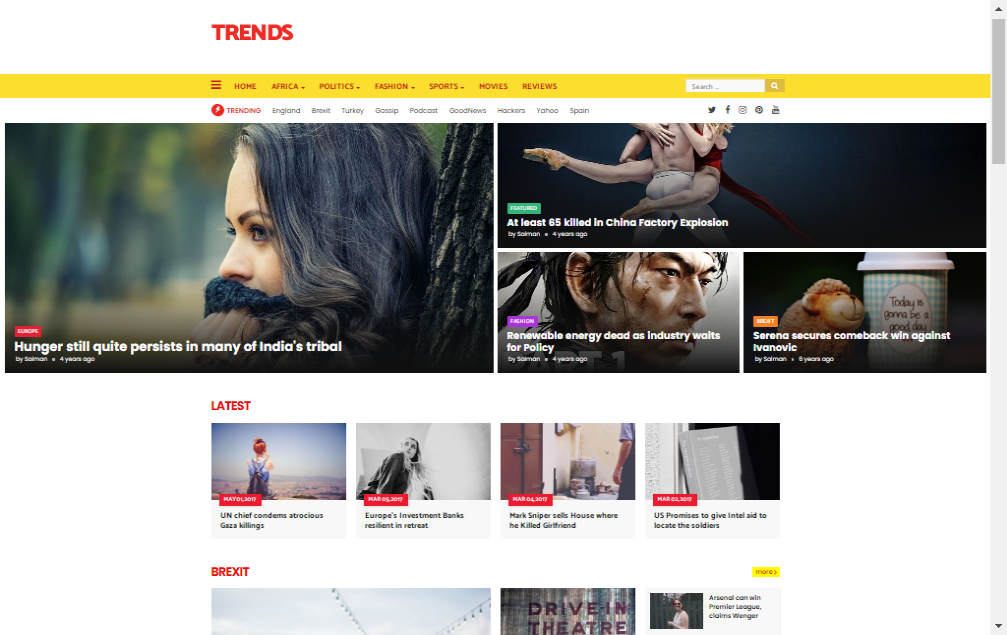This is a detailed website screenshot of the homepage of "Trends." The title "TRENDS" is prominently displayed in uppercase red font, located towards the upper left side but leaning slightly towards the center. Directly below the title, a yellow menu bar spans across the page, featuring navigation options in red font. From left to right, these options include "Home," "Africa" with a dropdown arrow, "Politics" with a dropdown arrow, "Fashion" with a dropdown arrow, "Sports" with a dropdown arrow, followed by "Movies" and "Review." On the far right of the same line, there is a search bar.

Further down, a white bar labeled "Trending" stands out, with additional menu options beneath it. One of these options, labeled "Funny," appears grayed out and is somewhat difficult to read. Below this menu section, there is a featured article titled, "Hunger Still Persists in Many of India's Tribes," accompanied by an image of a woman leaning against a tree. To the right side of this main article, there are more article options available for selection.